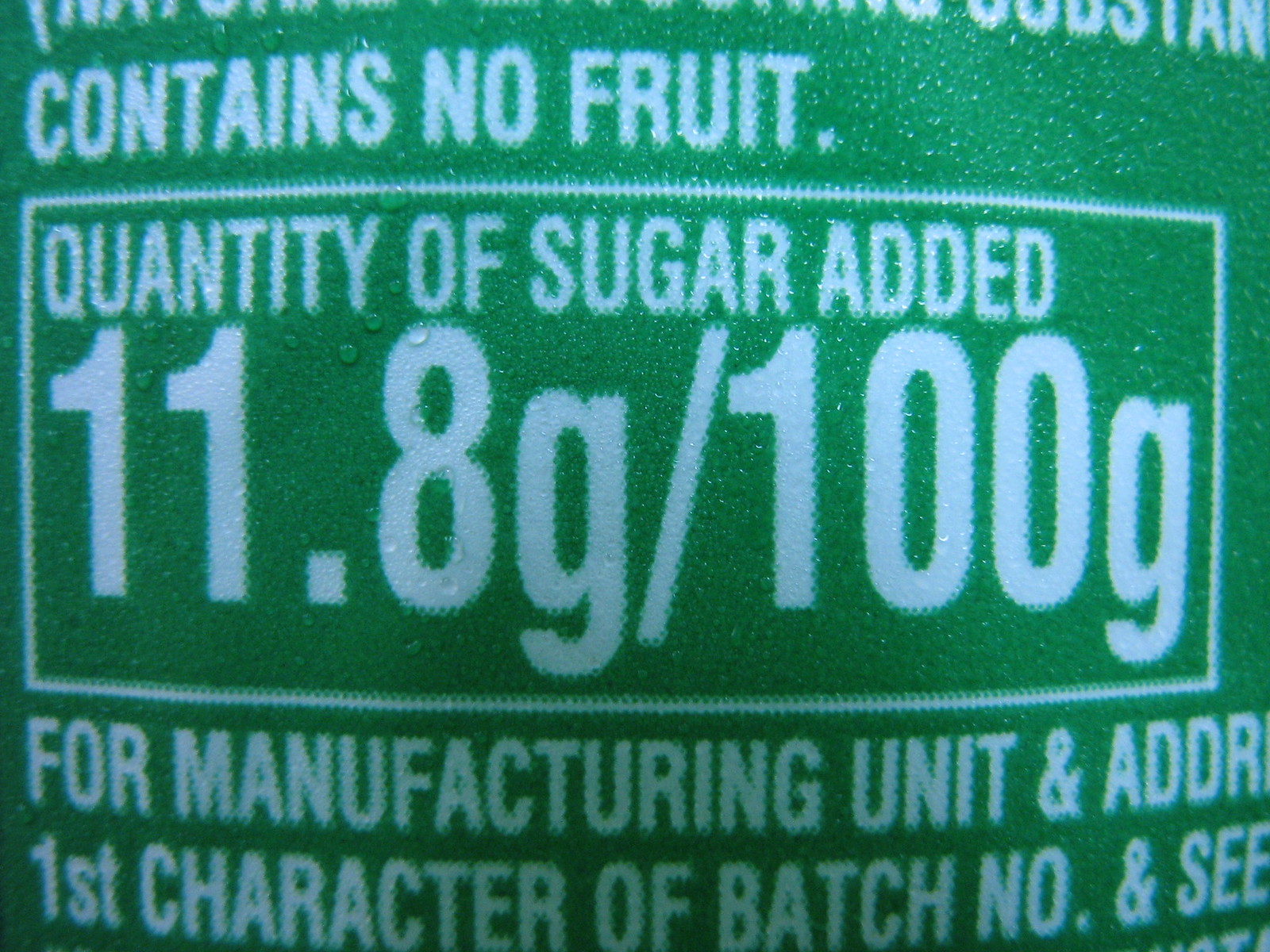This image showcases a highly zoomed-in, detailed view of a green can, likely a Sprite soda can based on the color. The can features white lettering, which is clearly visible against the green background. The most prominent text, enclosed in a rectangular box, states "quantity of sugar added 11.8 grams per 100 grams." Above this, another line reads "contains no fruit," written in white capital letters. Below the box, there is partially obscured text indicating information such as "for manufacturing unit and address," followed by "first character of batch number and SEE," although some words are truncated. The can has beads of condensation on its surface, suggesting it is cold and has likely been stored in a refrigerator.